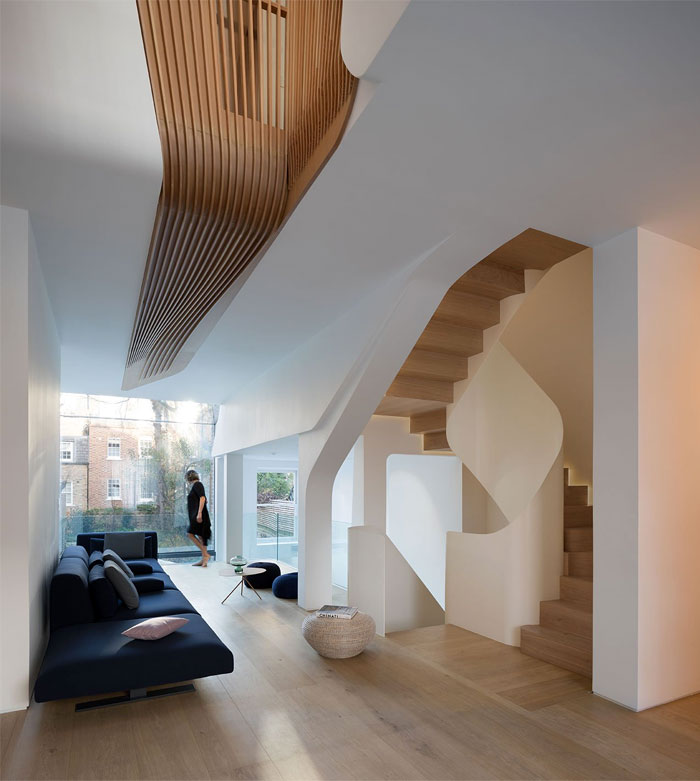The interior photograph captures a contemporary-styled living room characterized by its clean, minimalist design. The room features white walls without moldings, and light wood floors which add a warm touch to the modern aesthetic. Dominating the center of the space is a large, flat navy blue sofa that resembles a platform bed, adorned with several pillows. The room is illuminated by an expanse of glass windows that span one wall, offering a view of the buildings outside and flooding the space with natural light. There is a ceramic pot in tan and gray hues placed strategically, further enhancing the room's minimalist vibe.

The white, sleek staircase with matching white railings is situated at one end of the room, leading to the upper floors, and adding to the modern, open feel of the living space. Above, there are distinctive brown lines running across a portion of the angled ceiling, adding an interesting architectural element. Near the window stands a woman looking out onto the street, her presence adding a human touch to the serene setting. The room is also accessorized with a small table, contributing to the overall functional and stylish design.